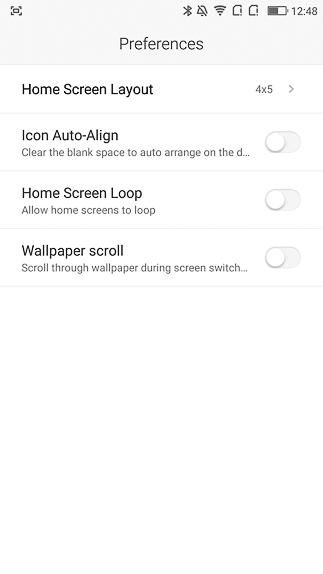This screenshot captures a detailed view of a user's Preferences page on their cell phone. The overall aesthetic of the image is minimalist with shades of white, black, and gray. Along the top edge of the screenshot, there are several icons and notifications, including the Wi-Fi symbol, battery life indicator, a bell icon with a line through it (indicating notifications are muted), and the current time, 12:48.

Immediately below these icons, the word "Preferences" is displayed on a light gray bar, setting the context for the options shown on the screen. The first visible preference is the "Home Screen Layout," set to a 4x5 grid, suggesting the arrangement of app icons on the home screen.

Three additional preferences are listed, each with a toggle switch, all of which are currently set to the off position:

1. "Icon Auto-Align": This option is intended to clear blank spaces by automatically arranging icons, though the descriptive text trails off: "clear the blank space to auto arrange on the D..."

2. "Home Screen Loop": Allows the home screens to loop continuously, making navigation more fluid.

3. "Wallpaper Scroll": Enables the wallpaper to scroll when switching screens, but its description is also incomplete: "scroll through wallpaper during screen switch..."

This screenshot provides a glimpse into the customization options available to the user, highlighting both the functionalities and the incomplete descriptions of certain features.